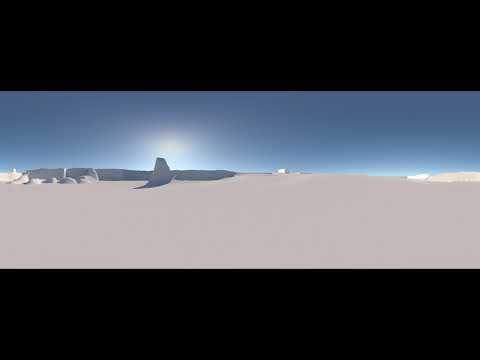A stunning, panoramic photograph captures a starkly beautiful desert scene in landscape orientation. The top half of the image is dominated by a brilliant, gradient blue sky, which darkens at the top and lightens towards the horizon until it almost merges with the white expanse beneath it. The sandy foreground stretches from left to right, resembling untouched snow with its smooth, pristine surface. Jagged edges of sand glisten on the left, while to the right, there appears a small pile of sand adding a touch of texture to the scene. Within this vast expanse of beige sand, a low, white-gray building punctuates the horizon, complete with a sharp upward projection toward its right side. Despite the clear presence of light illuminating the scene, no sun or celestial bodies are visible, giving an ethereal quality to the landscape. The top and bottom 10% of the image are bordered in black, framing the image and emphasizing the desert's isolation and serenity. No people or animals can be seen, underscoring the untouched, tranquil nature of this expansive desert vista.